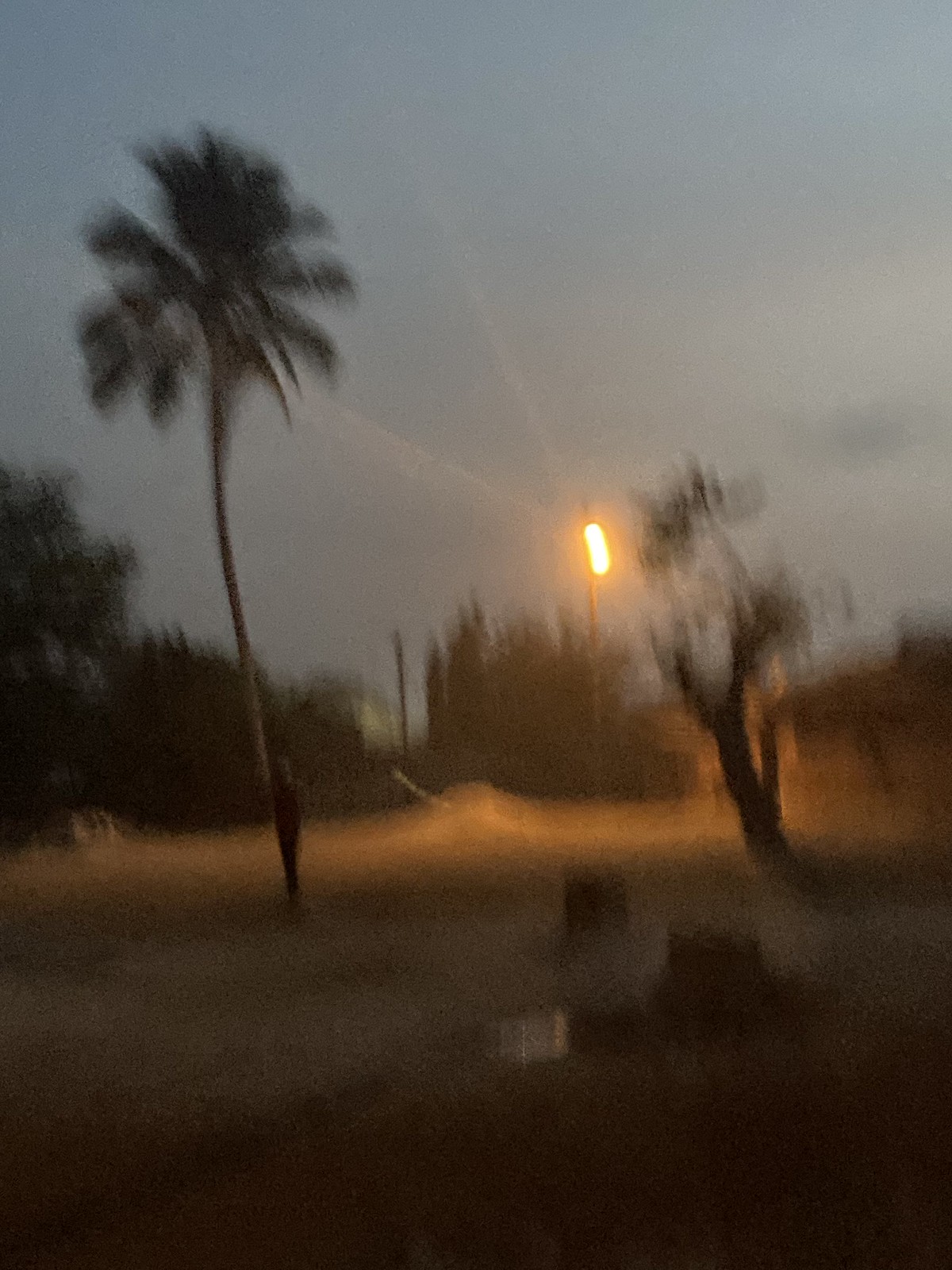Caption: 

In an unsettling, first-person perspective taken outdoors during the twilight hours, the blurry and fuzzy image conveys the motion of the photographer. A slim man stands eerily still on a grassy field adjacent to a footpath, separated by a sidewalk. He is positioned in front of a tall, slender palm tree, adding to the unsettling ambiance. To the right of the palm tree, a shorter but much thicker tree contrasts with its robust trunk. In the distance, a solitary street lamp casts a pervasive glow, contributing to the image's eerie atmosphere. The sky transitions from a light grey to a deepening dusk, heightening the overall spooky vibe of the scene.